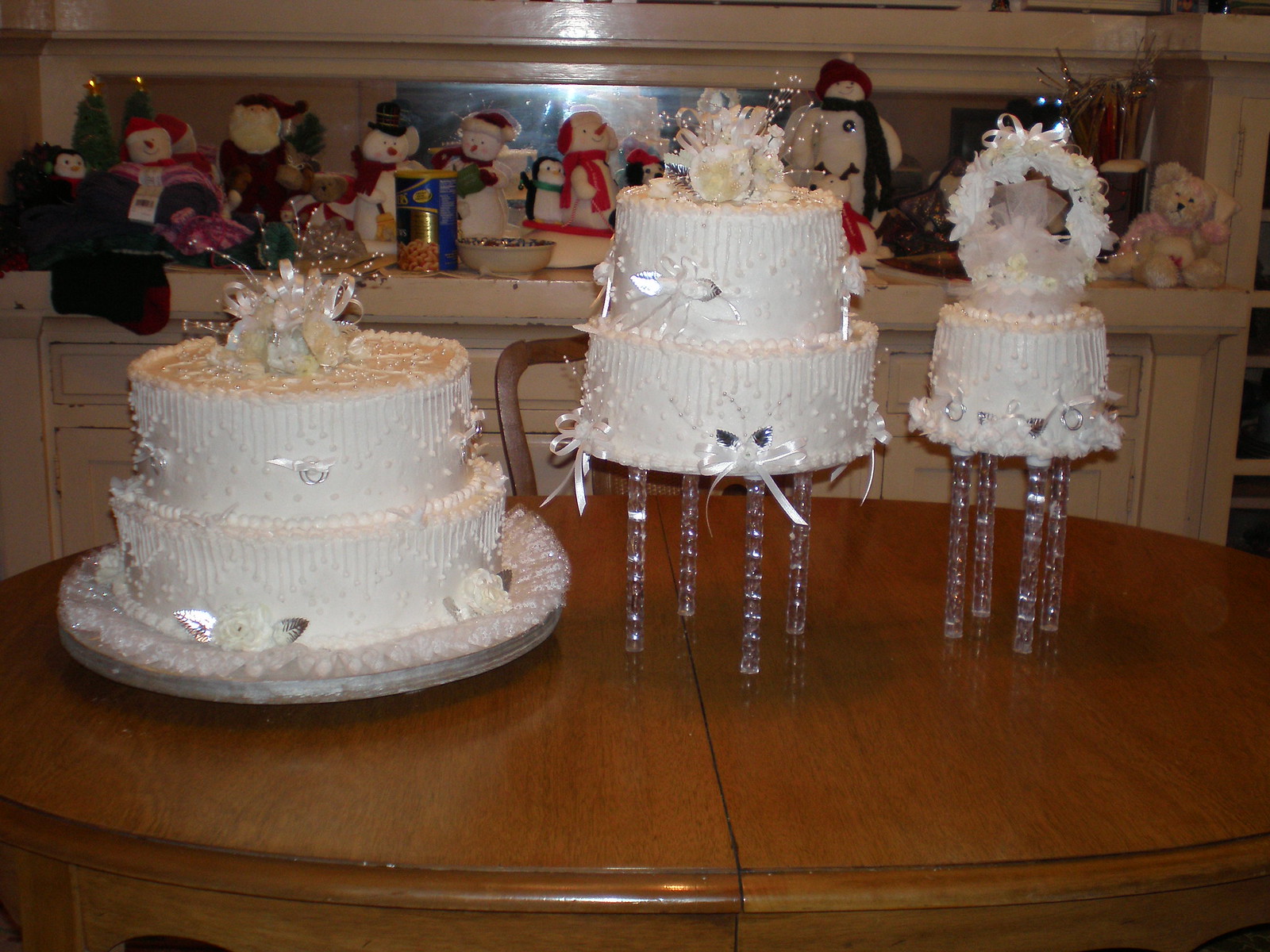This photograph showcases an elegant display of wedding cakes on a polished medium brown round table. The table features three cakes intricately arranged in layered tiers. On the left, the first cake consists of two layers, adorned with white icing, piped white flowers, silver leaves, and delicate plastic stamen sprays. This cake, placed on a cake plate, is topped with a floral arrangement featuring beaded sprays and roses.

Beside it, the second cake, also two-tiered but smaller in size, rests on a crystal pedestal with beaded legs. It is similarly decorated with white flowers, pink ribbons, and a white spray.

The third layer on the far right is positioned on another crystal stand and is crowned with a floral arch embellished with white ribbon and pink netting.

Behind the cakes, a white buffet cabinet adorned with festive decorations adds to the charm. The top shelf showcases figurines including a teddy bear, various snowmen, a Santa Claus doll, and Snoopy with a scarf, all reflecting a festive holiday theme. The setup exudes a blend of wedding elegance and cozy holiday cheer.